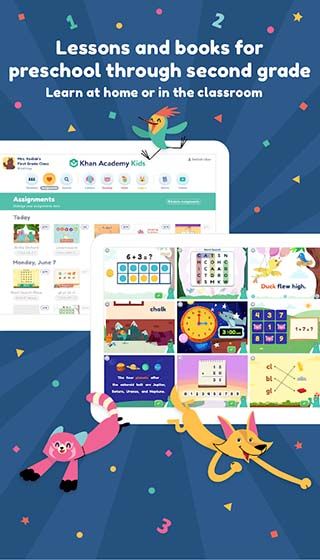The image, designed for mobile viewing, features a vertically-oriented screenshot with a captivating blue-striped background. These alternating blue stripes, varying from subtle dark to medium shades, radiate outward from the image's center, providing a vibrant backdrop. Scattered across the background are colorful and playful shapes—stars, squares, circles, and triangles—along with a few numbers, all in bright hues like yellow, red, purple, and blue.

At the top, bold white text reads, “Lesson plans for preschool through second grade. Learn at home or in the classroom,” setting an educational tone. Below this text, a trio of charming cartoon animals adds a whimsical touch: a jubilant green bird, a cheerful pink raccoon with black paws, and an elongated, happy yellow-brown dog.

The image also features two inset screenshots of the Khan Academy Kids app, each bordered in white. These screenshots showcase various educational activities aimed at young learners, including word searches and puzzles, designed to teach foundational skills like phonics.